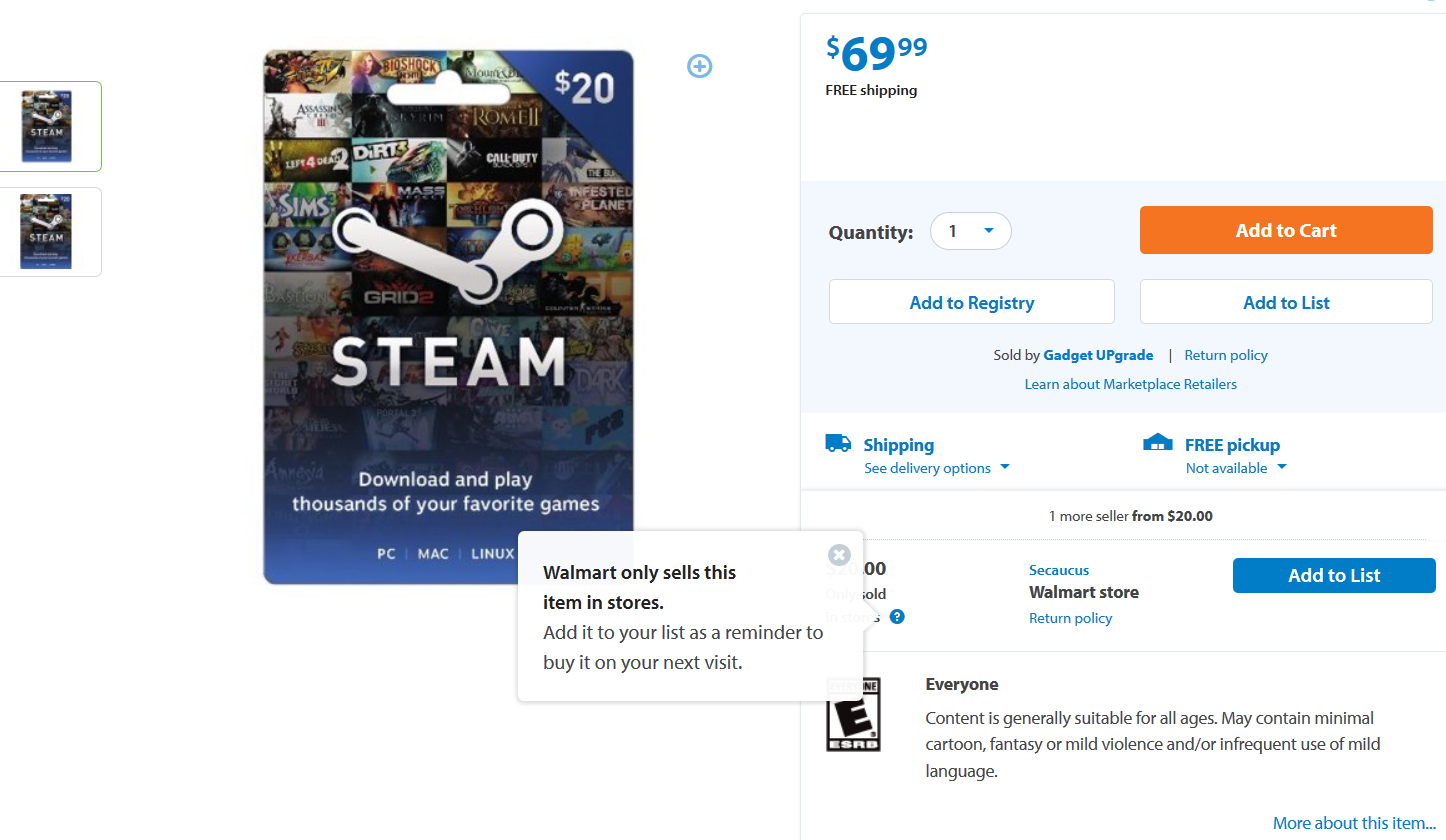This screenshot appears to be from an online shopping website, possibly advertising a gift card for the popular gaming platform Steam. The main promotional image, a vertical rectangle, prominently displays the Steam logo along with the text: "Download and play thousands of your favorite games." In the upper right-hand corner of the image, a price tag of $20 is visible, suggesting that this might be a Steam gift card.

On the right side of the screen, there is a section resembling an online store interface where users can make a purchase. An orange "Add to Cart" button is easily accessible, along with a selectable quantity drop-down menu currently set to 1. Below this, there are additional options to "Add to Registry" and "Add to List."

In the upper left-hand section above these options, the price is listed as $69.99 with free shipping available. Moving further down, below the "Add to Registry" and "Add to List" buttons, there is a shipping section. An icon next to the word "Shipping" provides a link to see delivery options via a drop-down menu. It also mentions that free pickup is not available and lists an alternative seller offering the item for $20.

The screenshot indicates that this item can be purchased at Walmart, including a link to Walmart's return policy. Lastly, it specifies that the game associated with this gift card is rated E for Everyone, indicating content generally suitable for all ages. This rating notes that the content may contain minimal cartoon, fantasy, or mild violence, and infrequent use of mild language.